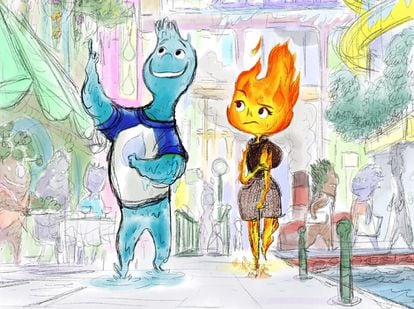This is a detailed, hand-drawn, color illustration showcasing two anthropomorphic characters inspired by elements, likely from the Pixar movie "Elemental." On the right is a female figure with a head of flames, complete with orange, yellow, and red hues resembling hair, and characterized by her feminine features, including expressive eyes with eyelashes, a small nose, and a partial frown conveying a puzzled expression. She is wearing a sleeveless brown top and light brown shorts, and her arms and legs are made of fire, trailing a little puddle of flames at her feet.

On the left, there is a taller, blue male figure reminiscent of a water droplet. He has spiky, water-like hair and a bright, cheerful face with black eyes and a wide smile. The water character is dressed in a white t-shirt with blue sleeves and a blue water droplet symbol on the chest. His right arm is pointing upwards toward the sky, and his legs are depicted as fluid, forming small puddles of water underneath.

The setting of the image is a bustling urban street scene. To the right of the frame, there is a small pool of water with people walking behind it, suggesting a busy city environment. To the left, there appears to be an area with a restaurant or café, indicated by a green awning and tables with people. The background fades into outlines of city buildings and possibly a subway entrance, adding depth to the scenery.

The overall style of the artwork is reminiscent of concept art or a movie sketch, possessing a pastel, watercolor-like quality. The image captures a moment where the two characters appear to be interacting, with the flame girl looking somewhat confused as she glances at the cheerful water guy gesturing upwards.